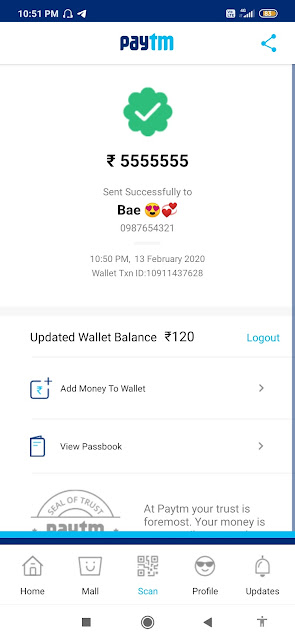The image captures a screenshot of an online transaction receipt from the PayTM application. At the top, the PayTM logo and the app's name are prominently displayed. Centrally positioned, a distinctive white checkmark over a green flower-shaped icon signifies a successful transaction. Below this icon, the message "5555555 sent successfully to Bae" is prominently displayed beside a smiley face emoji with heart-shaped eyes. The transaction details further specify that it occurred at 10:50 PM on February 13th, 2020. Additional information includes the Wallet ID and the updated wallet balance. To the right side of the screen, there's an option to log out. The interface provides two actionable buttons at the bottom: 'Add Money to Wallet' and 'View Passbook.' The background of the application is predominantly white. Notably, the current time, displayed in the top left-hand corner, reads 10:51 PM.